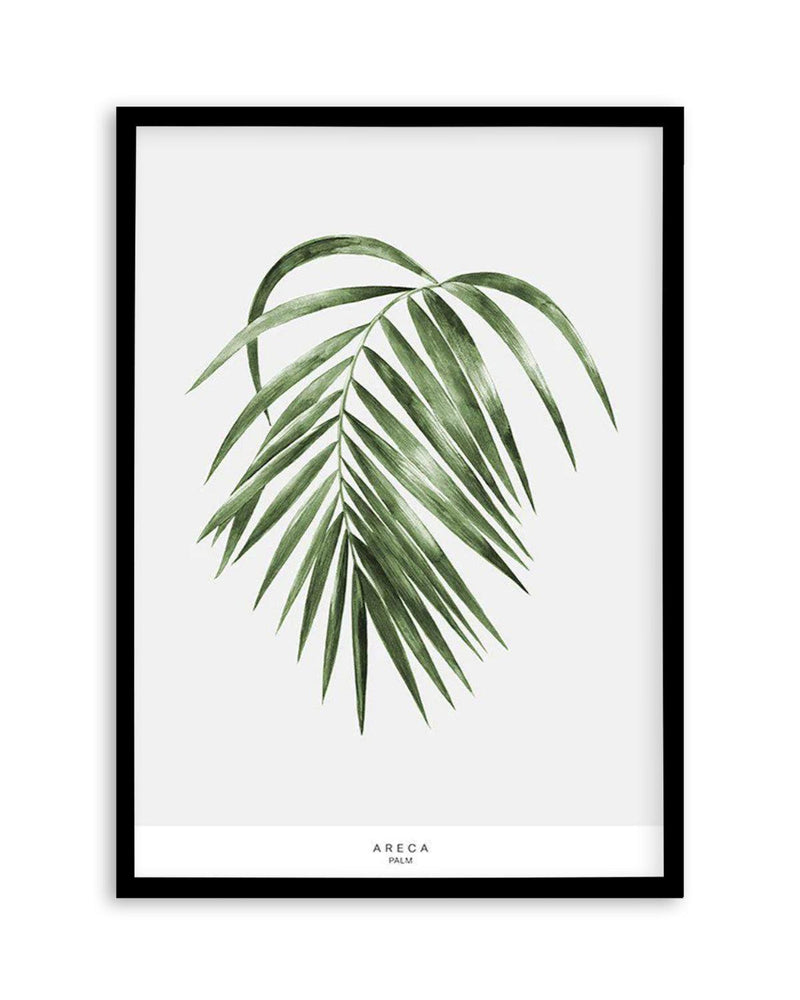This piece is a framed art print featuring a detailed illustration of an Areca palm leaf. The frame is thin and black, possibly made of metal, wood, or plastic. The print itself stands tall with a predominantly white background. The central focus of the artwork is a delicate green stem that begins in the upper right corner and curves gracefully down towards the center bottom. Extending from the stem are multiple long, thin, greenish leaves, fanning out symmetrically to the left and right. Towards the bottom of the print, there is a small white rectangle containing black text in spaced out, all-caps lettering spelling "ARECA PALM." The minimalist style and precise detailing make the Areca palm leaves the captivating focal point against the clean, light background.